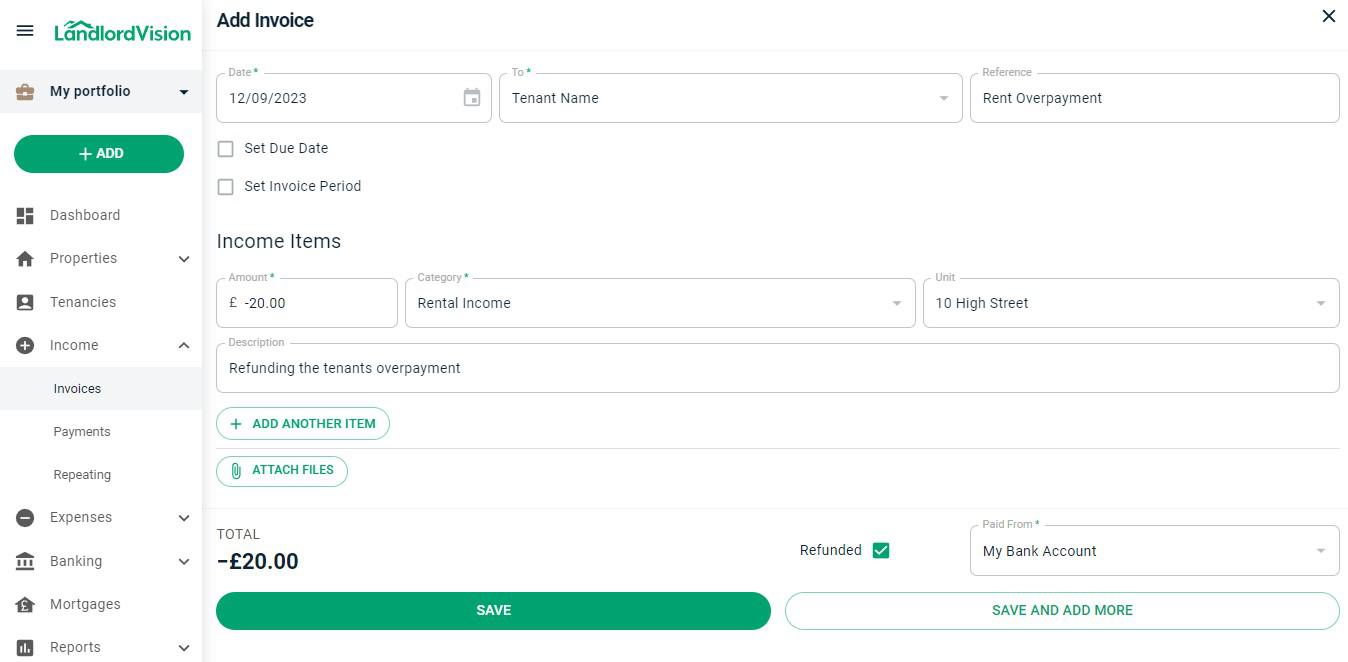This screenshot is taken from a website interface for a landlord management program called "Landlord Vision". At the top left corner, there is a black hamburger menu icon consisting of three horizontal lines. Adjacent to the right is the "Landlord Vision" logo, displayed in green font with a small house design creatively placed over the "AND" section of the word "Landlord".

On the left side of the screenshot, just below the logo, there is a vertical menu featuring various functionalities. Each menu item is accompanied by a corresponding icon. The menu items, listed top to bottom, include:

- Dashboard
- Properties
- Tenancies
- Income
- Invoices
- Payments
- Repeating
- Expenses
- Banking
- Mortgages
- Reports

On the right side of the screenshot, there is a section titled "Add Invoice". This section contains a form with multiple fields that need to be filled out. The fields include the date, tenant name, rent overpayment, and income items, with specific slots to input additional details.

At the bottom of this invoice form, there is a summary displaying a total of minus 20 Euros. Below this summary are two buttons: a green button labeled "Save" and, to its right, a white button with green text that reads "Save and Add More".